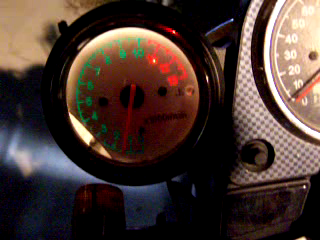The image depicts two distinct gauges set against a gray and white checkered background, possibly part of an old-fashioned instrument panel. The first gauge is designed with a dark face and features a lime green scale numbered from 1 to 10. Its orange needle stands out prominently, and it is adorned with three small orange symbols. Adjacent to this gauge is a classic speedometer, showcasing a black exterior and a white inner ring. The speedometer scale ranges from 0 to at least 80, though it likely extends beyond that. It has white numbers and a red needle. The overall setting is accented with shades of blue and beige, providing a subtle color contrast to the predominantly monochromatic gauges. Notably, there is no writing or additional text present on either gauge, allowing their visual elements to speak for themselves.